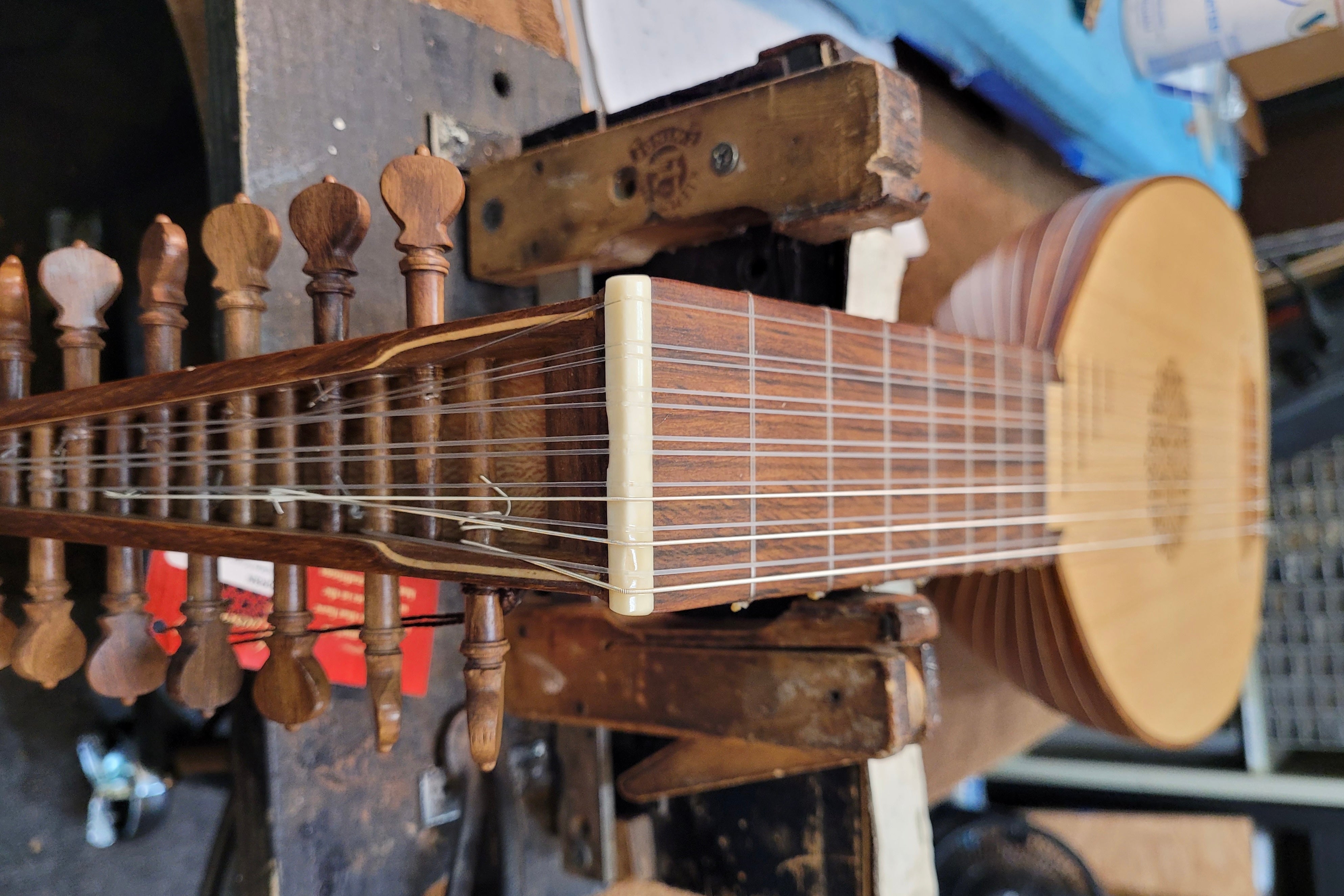The image depicts a unique stringed instrument that closely resembles a non-traditional guitar, featuring two interconnected necks. The body of the instrument transitions from a light yellow wood on the upper section to a darker brown decorated with a swirl pattern on the lower section, resembling the texture of an open coconut. The right side of the base features a small, dark brown circle. The necks are dark brown with numerous white strings stretching upwards, intersecting a white line before extending back down along a lengthy wooden section equipped with adjustment knobs, or tuning pegs. These knobs allow for the tightening and adjustment of the strings, which appear either white or clear and are visibly tied to the pegs. The entire instrument is mounted in a clamp, indicating it is being worked on, possibly in some sort of shop, and is suspended in mid-air against a wooden backdrop.